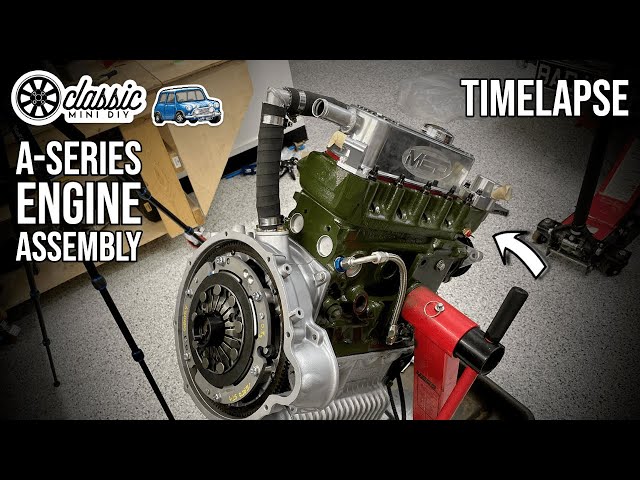The image appears to be a letterboxed screenshot of a video, likely an advertisement showcasing engine assembly. A black band runs across the top and bottom of the image. Dominating the center is a detailed photograph of an A-Series engine with a green body, supported by a red professional jack on a workshop floor. Surrounding the engine are various components, indicating a busy workshop environment. On the left side of the image, there's a logo featuring a spoked wheel and the text "Classic Mini DIY" in a script font, accompanied by a small image of a blue Mini car. Below this logo, the text reads "A-Series Engine Assembly" in caps. On the right side, an arrow points to the engine with the caption "Time Lapse" highlighting the video’s nature. A wooden worktable is visible in the upper left corner, further emphasizing the workshop setting.